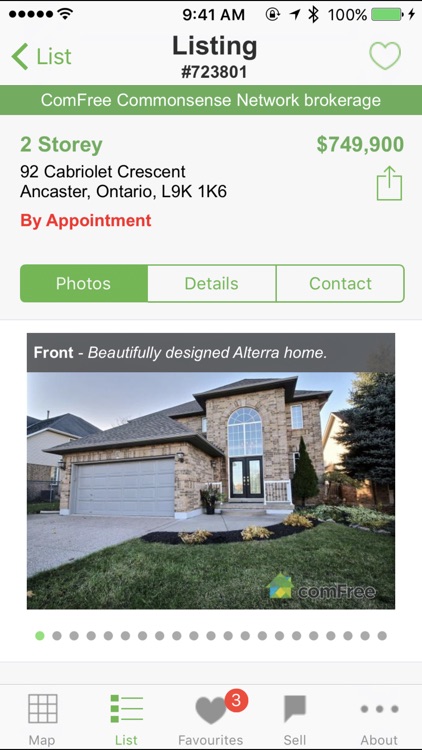**Detailed Caption:**

This image is a screenshot taken on a smartphone of a property listing on a real estate website. The phone’s status bar at the top shows a service indicator, the time at 9:41 AM, a Bluetooth indicator, and a fully charged battery icon indicating it is currently charging. The main content displays listing number 723801 with navigational buttons, including a back button to the left and a heart-shaped favorite button to the right.

The property is listed by Compre Common Sense Network Brokerage and features a two-story home located at 92 Cabriolet Crescent, Ancaster, Ontario, L9K 1K6, priced at $749,900. The listing notes that viewings are by appointment only. Below the property details, there are buttons for "Photos," "Details," and "Contact," with the "Photos" section currently selected.

The screenshot highlights a photo gallery showing the first image captioned, "Front Beautifully Designed Altera Home." The image showcases the front exterior of the home featuring stonework walls, a well-maintained front lawn, and a driveway. Additionally, there is a watermark in the lower right corner of the photo that reads “Compre” alongside a house logo.

At the bottom of the screen, there are five navigation buttons labeled "Map," "List," "Favorites," "Sell," and "About," providing additional functionality for browsing and managing listings.